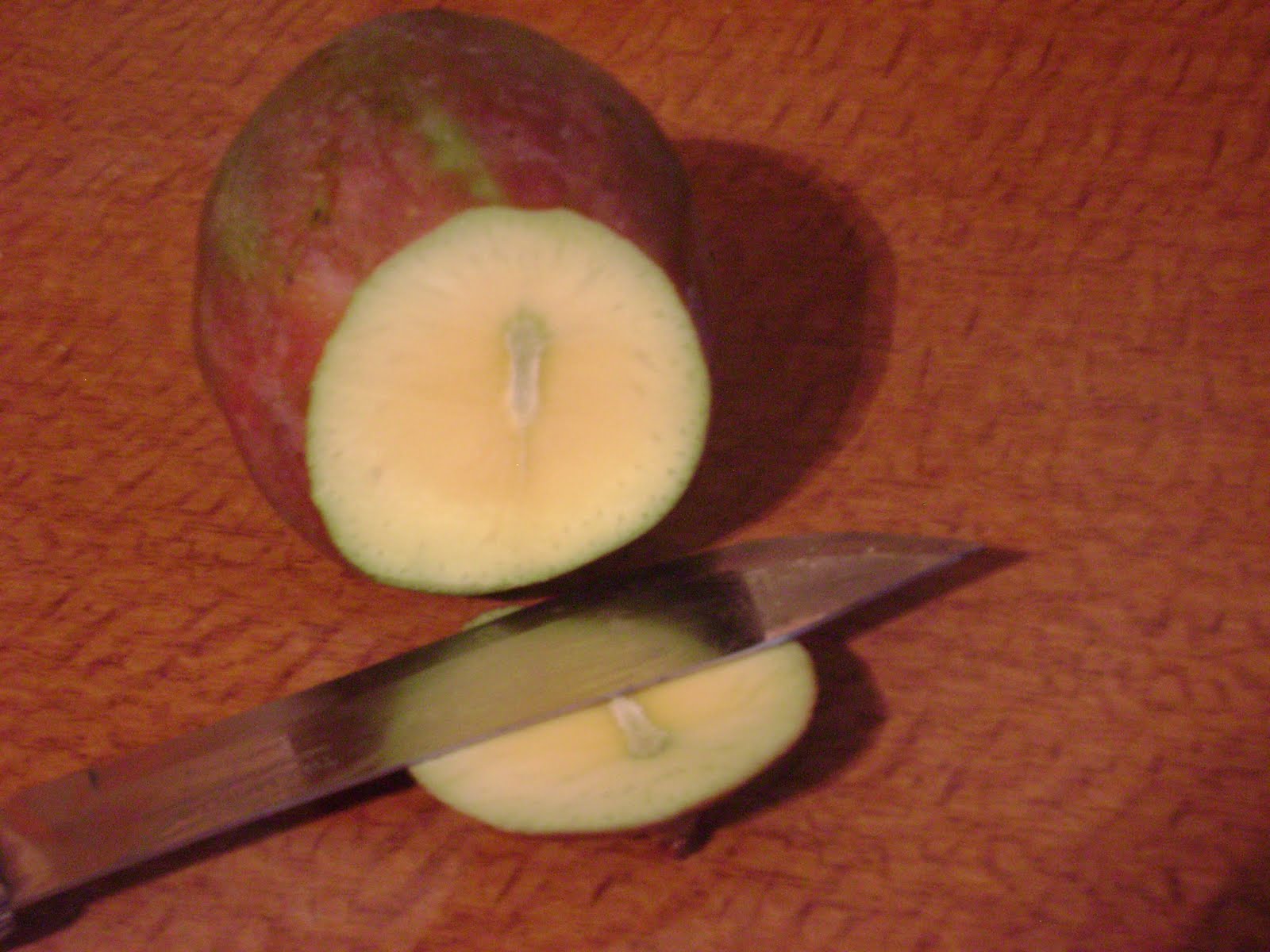The image displays a red apple with small green stripes on one side, set on an orange countertop with faint dark patterns. A segment of the apple has been cut off, revealing a light cream-colored interior with a lighter, possibly moldy portion at the center. The cut segment has a green border and a slit with white flesh. A well-used, sharply pointed silver knife, reflecting the apple's interior on its blade, lies atop the apple slice. The overall scene feels old-fashioned and somewhat unappealing.